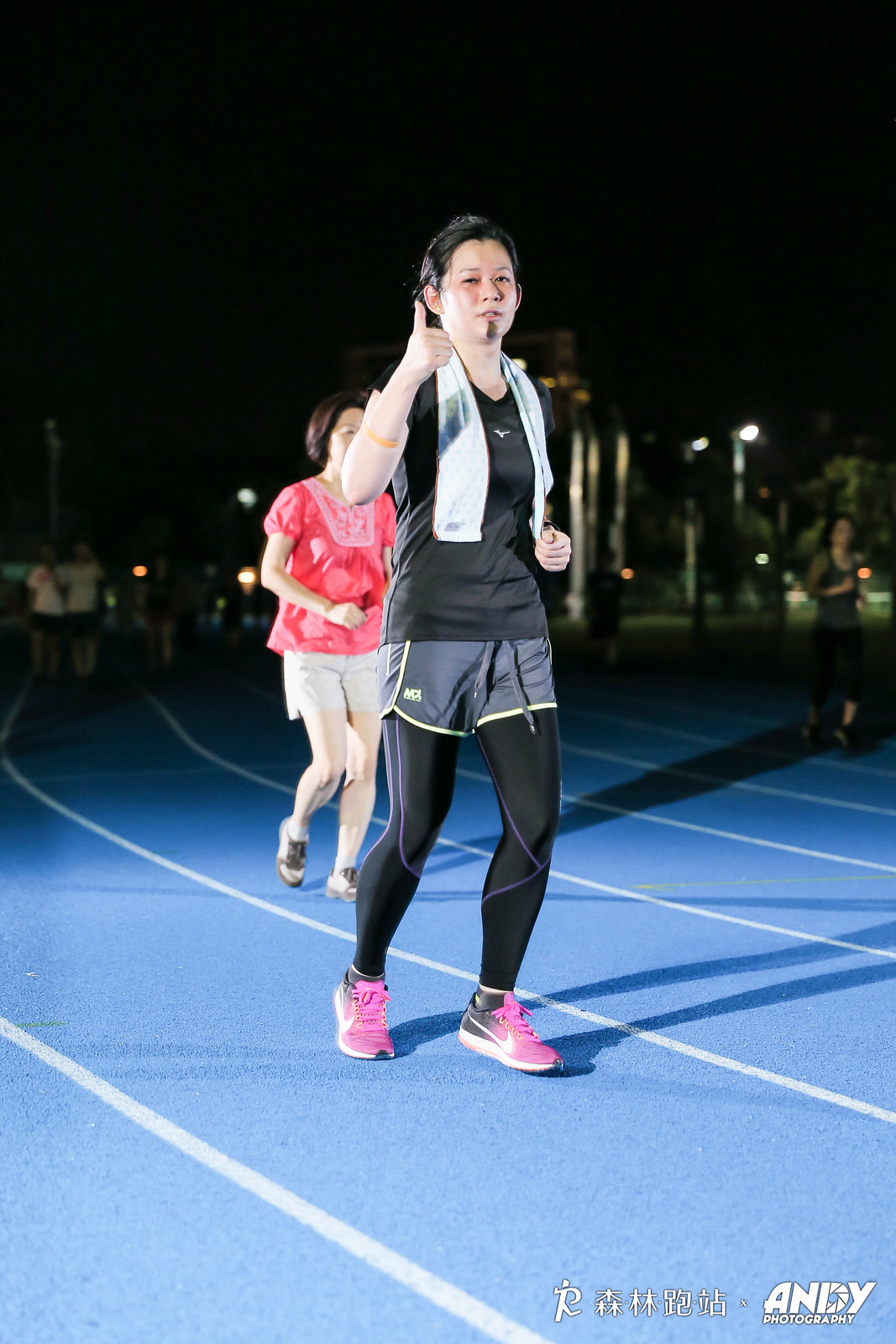The nighttime photo captures a woman running or walking on a blue track with white lines. She wears a black T-shirt, gray workout shorts with white trim, black tights, and pink Nike sneakers. A white towel is draped around her neck, and she has short black hair. She gives a thumbs-up gesture, facing the camera, while a mysterious black line runs from beneath her lips to her chin. Illuminated from the side, the track and nearby runners cast long shadows. In the blurred background, streetlights and additional runners are visible, including a woman in a red shirt and color shorts seemingly in motion. The dark sky and the artificial lighting add a dramatic ambiance to the scene.